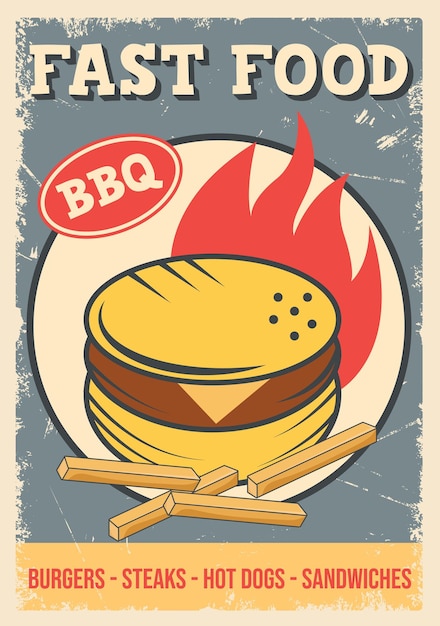This vintage-style fast food restaurant advertisement features a worn, beige-bordered sign reminiscent of the 1960s or 70s. The central part of the image is dominated by a blue rectangle with a yellow section at the bottom. At the top, large block letters spell out "Fast Food" in white with a subtle shadow effect. Just below, in the top left corner of a prominent central circle with a navy blue border, there is a red oval containing the text "BBQ" in white. Inside this circle, a cartoon cheeseburger with visible cheese, a bun, and a meat patty takes center stage, accented by flames in the background to indicate it's freshly grilled. In front of the burger, four French fries are scattered at different angles. The bottom yellow section contains a list of menu items: "Burgers - Steaks - Hot Dogs - Sandwiches," written in bold red text. The colors are deliberately muted, adding to the ad's nostalgic and aged appearance.